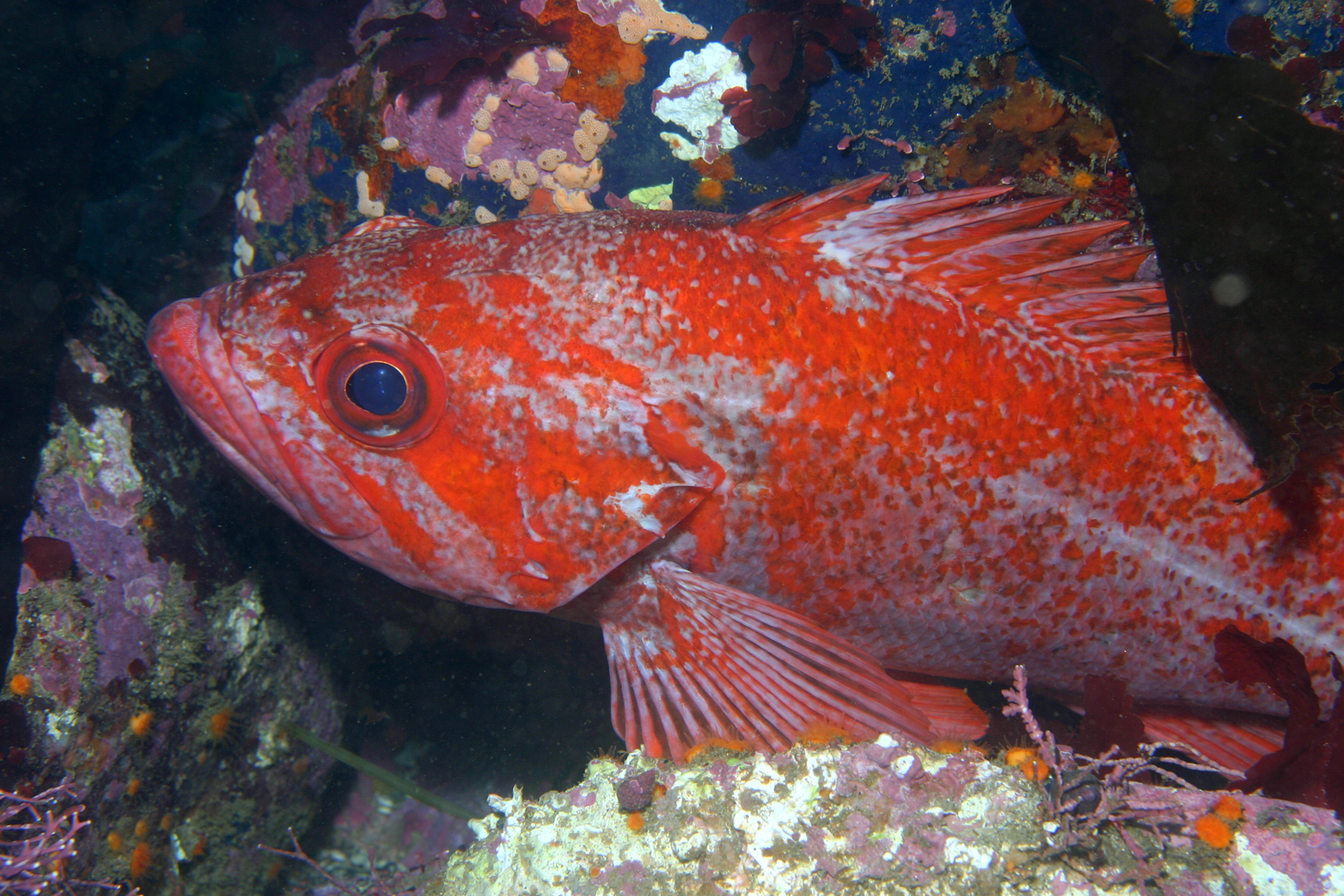This image features a close-up view of a vibrant, tropical fish in an aquarium setting. The primary subject, a predominantly orange fish with mottled white and silver spots, appears to have a textured, almost chipped look to its color. Its large, black eye gazes towards the left side of the frame, with a spiky dorsal fin and fins at the bottom. Although we can't see its tail, the fish's body is visible from the side. The aquarium surroundings, consisting of colorful rocks and a few patches of purple coral-like formations, suggest an artificial habitat rather than a natural underwater environment. The ground is covered with typical aquarium pebbles, some of which show hints of green moss. No other fish or vegetation are visible in the image.